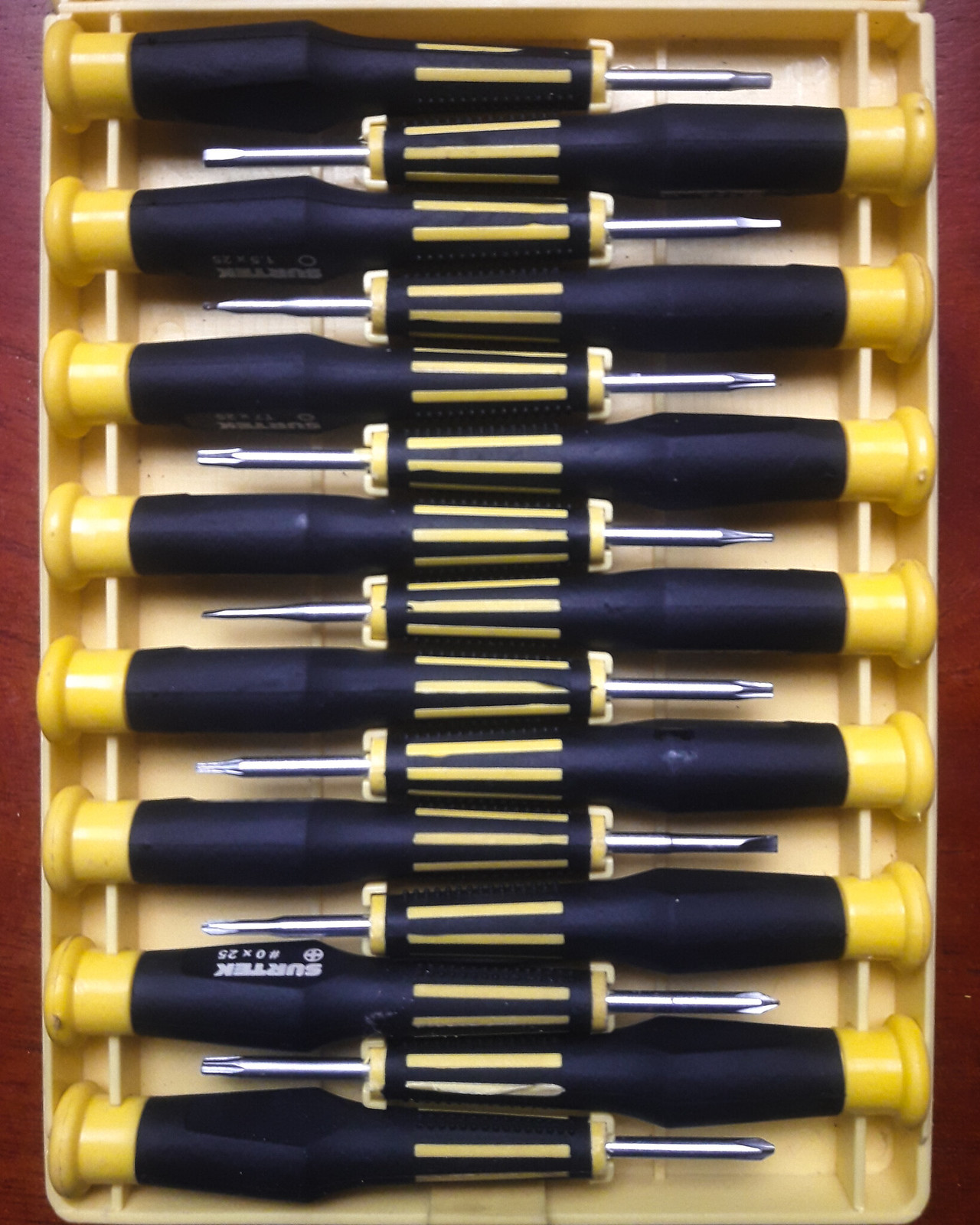The image features a detailed photograph of a set of 15 screwdrivers arranged in a yellow plastic case. The screwdrivers, which include flathead, Phillips, Torx, and square types among other specialty precision screwdrivers, have black handles with yellow flat tips. The handles also feature black and yellow striped patterns near the base, leading to short metal shafts. Each screwdriver has a silver plastic washer near the metal part, adding a touch of contrast. The screwdrivers are meticulously organized in the case, alternating direction with the handles on the left for one, right for the next, and so on. This alternating arrangement fits perfectly within the slots of the rectangular case, which itself is oriented vertically in the image. The entire setup rests on a wooden surface, and it appears the case is encased in a wooden box, enhancing the presentation. The brand name, which starts with an 'S', is partially obscured and hard to read, adding a slight mystery to this well-kept tool collection.